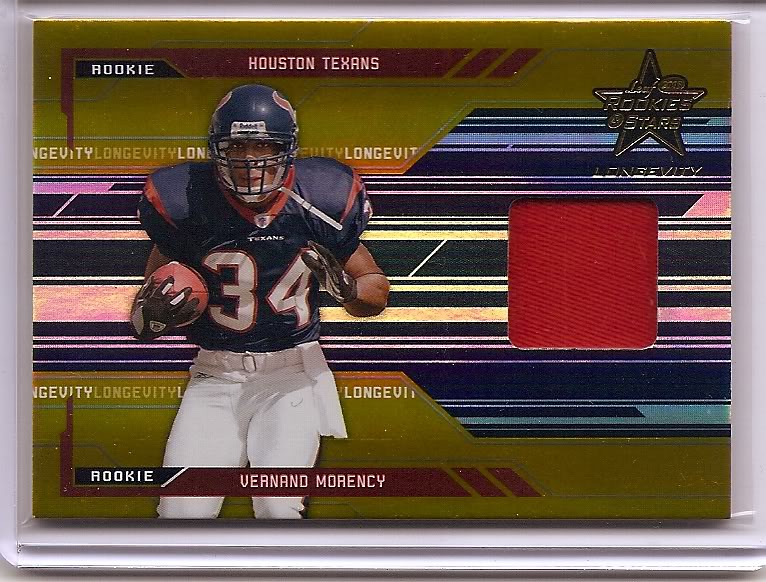This image is of a commemorative football card in a plastic sleeve, showcasing a rookie player from the Houston Texans. The card predominantly has a gold background with a thin white plastic border on all sides. Across the top left corner, there's a black box with the word "Rookie" followed by "Houston Texans." In the upper right corner, there's a star that reads "Rookie Stars Longevity." The card features a football player in full gear standing in the left center of the image. He wears a blue Houston Texans jersey with red accents, white football pants, dark gloves, and a blue helmet with red accents. His jersey has the player number 34, and he is cradling a football between his right hand and right bicep, with his left hand extended forward. At the bottom of the card, there's a black bar with the text "Rookie" and next to it the name "Vernand Morency" in white letters. To the right of the player, there's a red square, which might be a design element or a piece of the jersey.